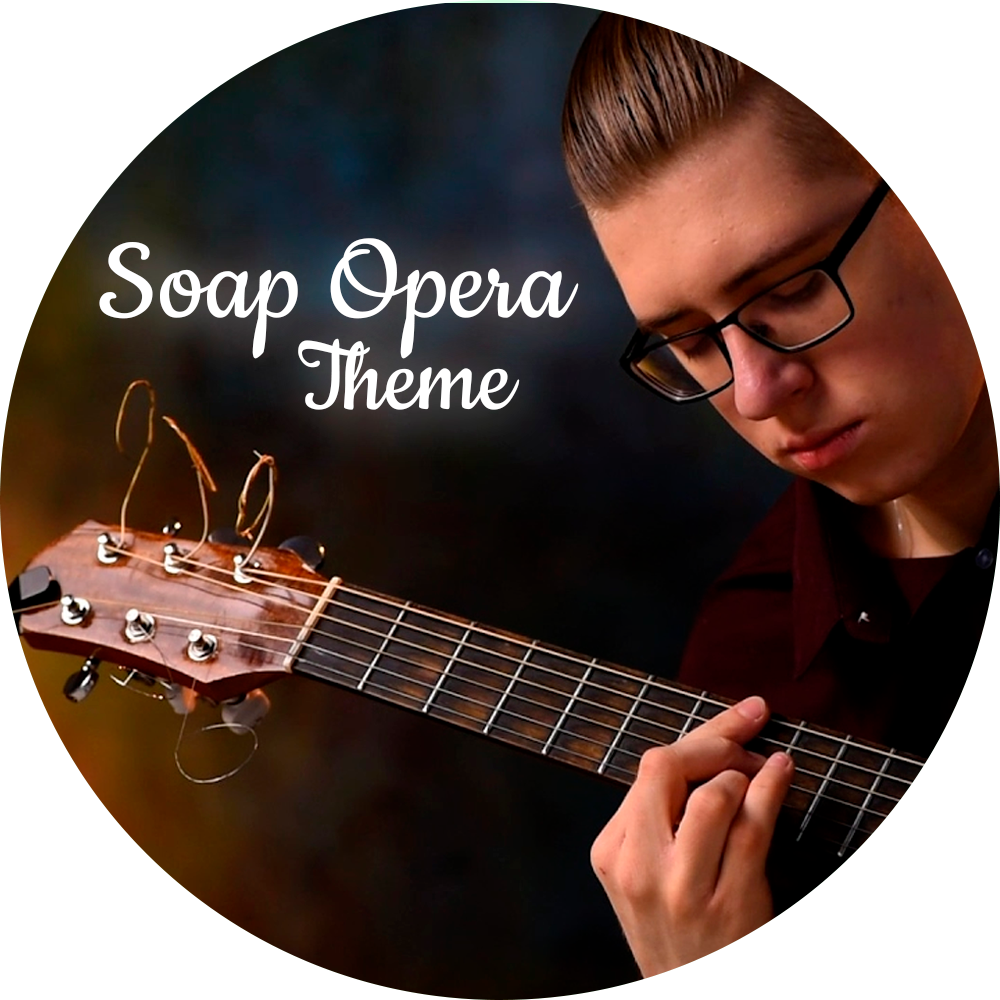The full-color circular photograph, professionally staged and shot for a promotional purpose, features a young Caucasian male playing a guitar indoors with artificial lighting. The background is out of focus, possibly showing a gray curtain or wall with a touch of orange on the left side. The man's brown hair is slicked back, and he wears black glasses and a black outfit, accessorized with a necklace. His eyes are closed as he hits a note on the guitar, which has loose, curly strings sticking out from the neck. The white cursive text at the top left of the image reads "soap opera theme."